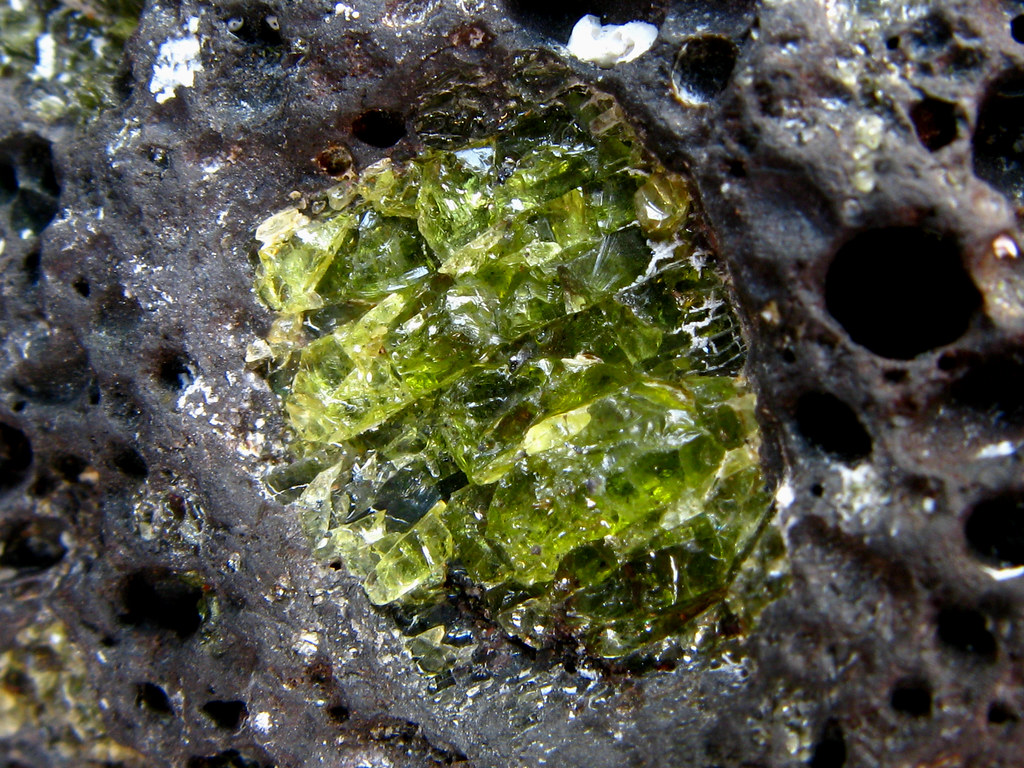The image is a detailed close-up photograph capturing a vibrant green gemstone embedded within a dark, charcoal gray rock. The gemstone, located centrally, displays a jagged and unpolished surface with sharp edges, enhancing its rough and natural appearance. Its glassy green hue reflects an overhead light, possibly natural or artificial, making it shine and stand out against its contrasting surroundings. The encasing rock has a cement-like texture, marked by numerous pockmarks and craters, giving it a spongy yet solid look. The left upper quadrant of the rock shows a hint of a similar green color, while the right side transitions more into gray and black tones, adding depth and complexity to the scene.